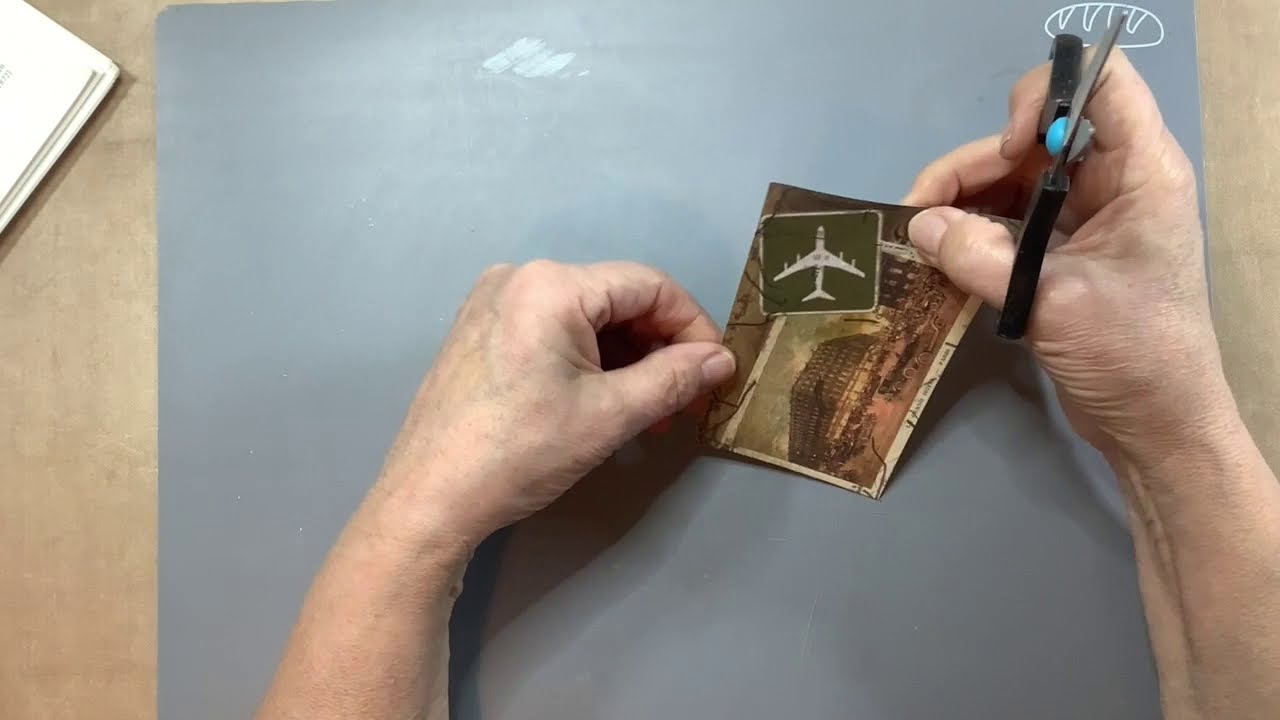The image depicts a pair of white hands above a gray surface, likely working on a craft or project. The individual's right hand, identifiable by short fingernails, holds a black-handled pair of scissors with a distinctive blue dot near the pivot. Both the thumb and middle finger of this right hand are also gripping a card or photo.

The card depicts a brown multi-story building with a white jumbo jet featuring long wings and four engines positioned diagonally above it. In the upper right corner of the card is a drawing resembling a loaf of bread with slits on top. The surface beneath the hands is gray, contrasting with a brown base underneath it. In the upper left corner of the image, part of an open white book is visible. The background includes light blue tones, possibly featuring an abstract cloud or cave-like illustration. Various participants have noted the card may have writing at the bottom, further adding to the complexity of the scene.